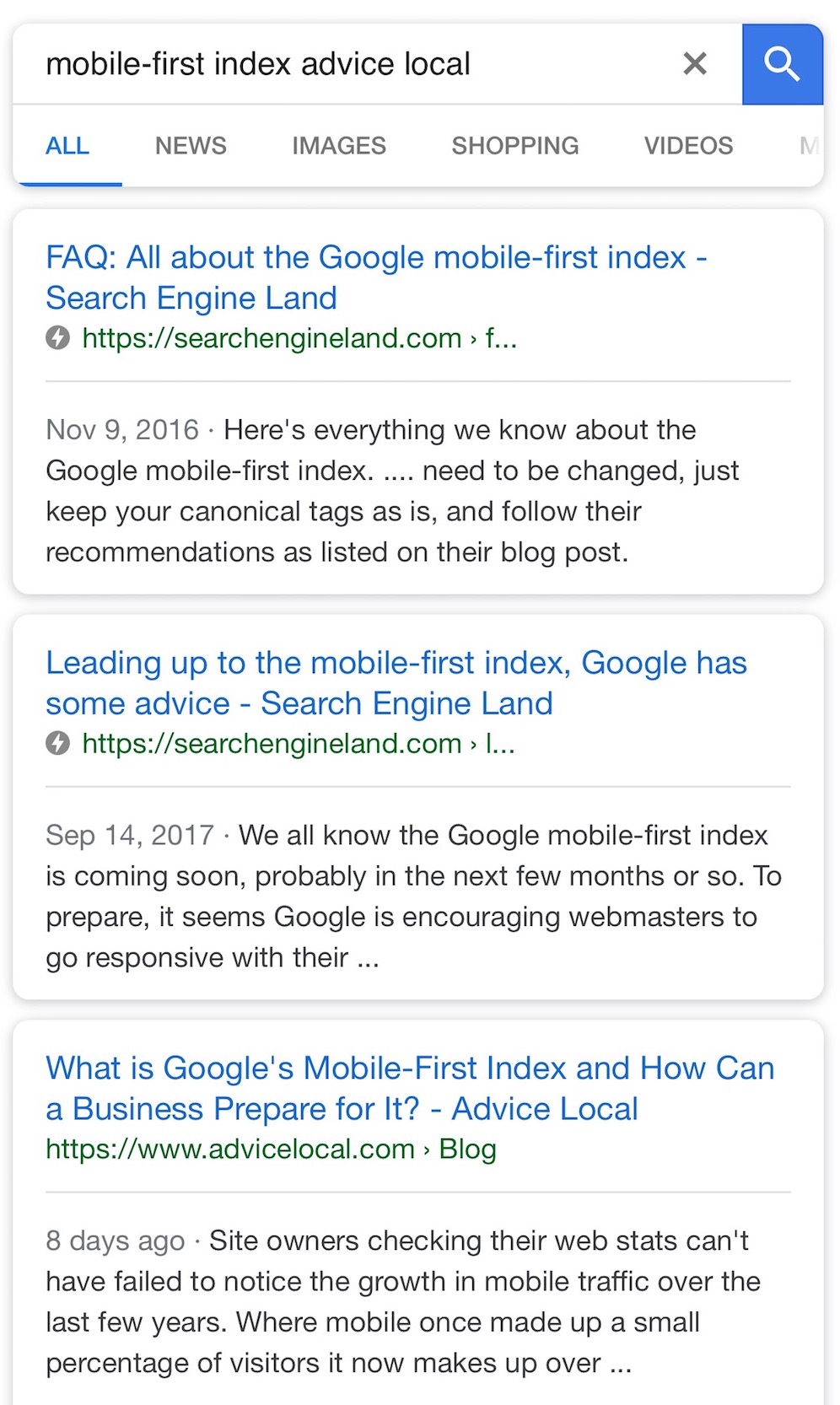The image depicts a section of a website with a clear, detailed layout. The background is predominantly white. At the top of the webpage, there's a search box positioned centrally, featuring an 'X' icon on its right side and a blue rectangular button with a search icon to the far right.

Below the search box is a line of navigation tabs. The first tab is highlighted in blue, indicating the currently selected category, while the remaining tabs appear in black. The tabs are labeled as follows: "All," "News," "Images," "Shopping," and "Videos."

Beneath the navigation tabs is a prominent FAQ section about Google's mobile-first index. The title of this section, “Google Mobile First Index: What You Need to Know,” is prominently displayed in blue text. The associated URL, "https://searchengineland.com," is shown in green, accompanied by an 'F' and three dots icon. 

The first result is titled "November 9th 2016: Everything We Know About Google Mobile-First Index" and discusses the importance of keeping canonical tags unchanged and following specific recommendations from a referenced blog post.

Following this, there are two additional search results presented in a similar format:
1. "Leading Up to the Mobile-First Index: Google Has Some Advice," from the same website, Search Engine Land.
2. "What is Google's Mobile-First Index and How Can a Business Prepare for It?" from the website Advice Local, posted eight days ago.

The snippet of text under the second result emphasizes the dramatic increase in mobile traffic over the years, noting that while mobile traffic used to be a minor portion of overall visitors, it has now grown significantly.

Each result is structured to provide useful insights about Google's mobile-first indexing and how businesses can adapt to these changes.